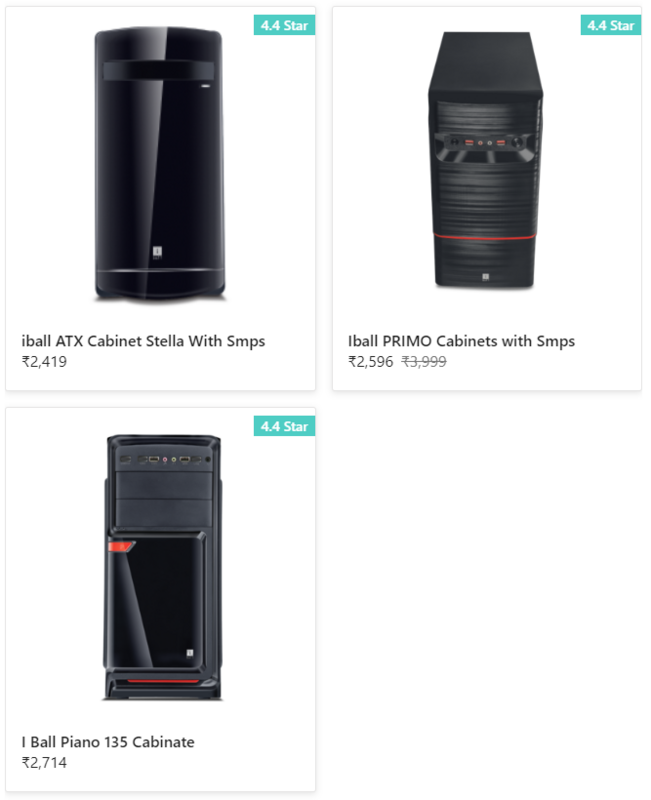This image, set against a solid white background, displays three products for sale, each set within a gray outlined box. The first product, located in the top left corner, is a rectangular black item labeled "Eyeball ATX Cabinet Stella with SMPS." It is priced at $2,419 and carries a rating of 4.4 stars, which is displayed in white text on a mint green box in the upper right corner. Directly beneath this, another rectangular black item appears with a similar design and a 4.4-star rating in the upper right corner. Below it, the product is identified as "One Ball Piano 135 Cabinet," priced at $2,714. The final image in the bottom row shows another product tagged as "Eyeball Primo Cabinets with SMPS," listed at $2,596 and also rated 4.4 stars, highlighted within a mint green box in the upper right corner.